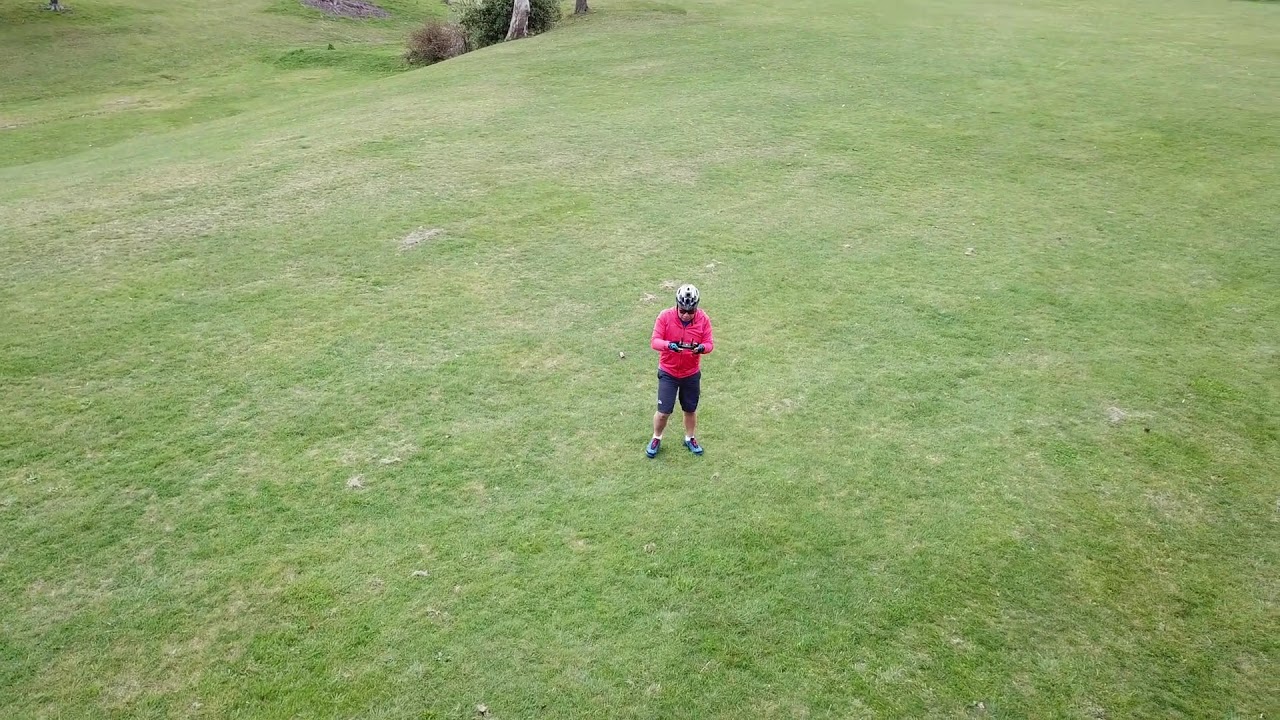This aerial photograph, taken approximately 20-25 feet above ground, showcases a man standing in the middle of a large grassy field. The man is wearing a bright red shirt, black knee-length shorts, and light blue sneakers with white ankle socks. He also sports a white bicycle helmet and glasses. In his hands, he holds a black joystick device, indicative of controlling a drone from which this image is likely captured. He is the sole individual in the image, and his focus is on the controller. The expansive green field around him is mostly uninterrupted, with the exception of some tree trunks near the top edges and a few scattered bushes. The terrain subtly inclines, particularly on the upper left side, where a drop to a lower level of grass can be observed, along with a bare patch in the greenery.